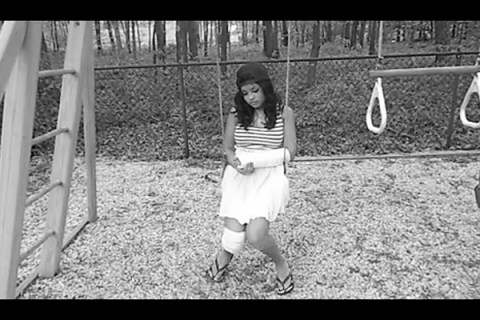This black and white photograph captures a somber moment of a young woman sitting on a playground swing, the focus of the image. The scene is bordered by black bars at the top and bottom of the frame, adding a cinematic feel. On the left side, a ladder of a play structure extends from the bottom left to the top left of the frame. To the right, part of a swing set is visible, with two white handles hanging down. 

Central to the image, the woman sits on the swing with its strings coming down from the top of the frame. She is dressed in a dark and white striped tank top, a white skirt that ends above her knees, and dark flip-flops. Her long dark hair flows past her shoulders, contrasted by a black baseball cap worn backwards. Her gaze is cast downward, her expression reflecting sadness. Both of her hands are clasped together in front of her, revealing a bandage on her left arm and another on her right knee. 

Behind her, a dark chain-link fence delineates the boundary of the playground, beyond which a dense, dark wooded area looms. The mix of playground elements and the woman's pensive demeanor create a poignant, evocative scene.